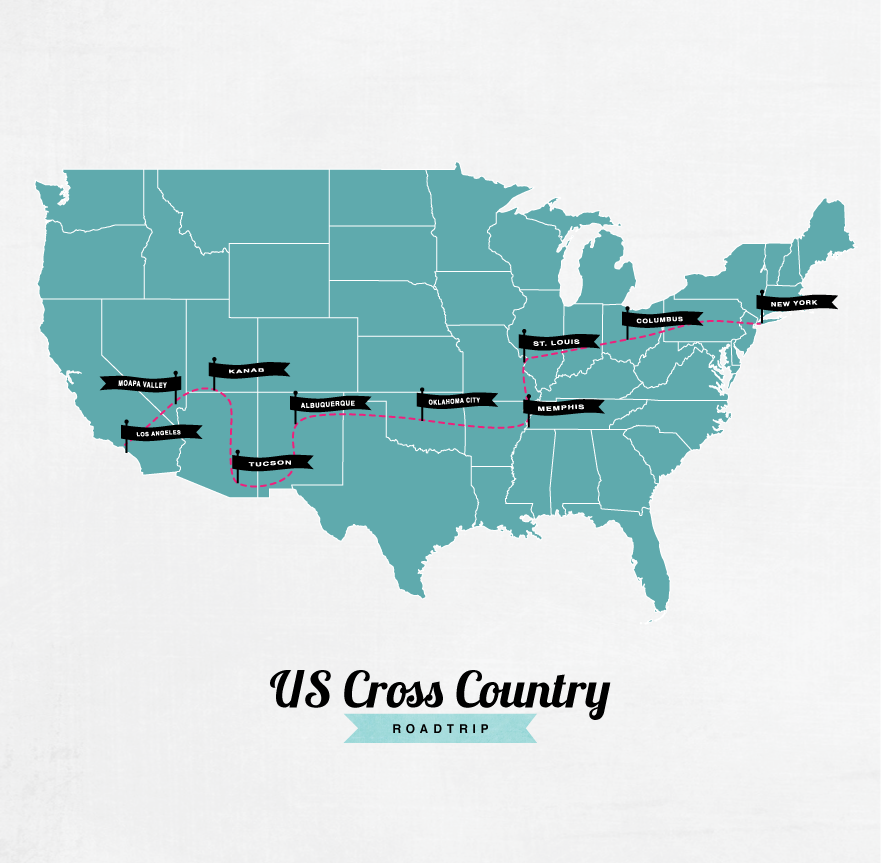The image is a detailed map of the continental United States mounted on a light gray background. The map is teal in color with white lines delineating each of the 48 states. The bottom of the map features the title "U.S. Cross Country Road Trip," with "U.S. cross country" written in black and "road trip" in a teal flag. A red dotted line traces a cross-country route from Los Angeles to New York, passing through several key locations marked with black flags labeled in white. These flags highlight the stops: Los Angeles, Moapa Valley, Tucson, Albuquerque, Oklahoma City, St. Louis, Memphis, Columbus, and New York. The map is devoid of any other markings, focusing solely on the outlined states and the cross-country journey.